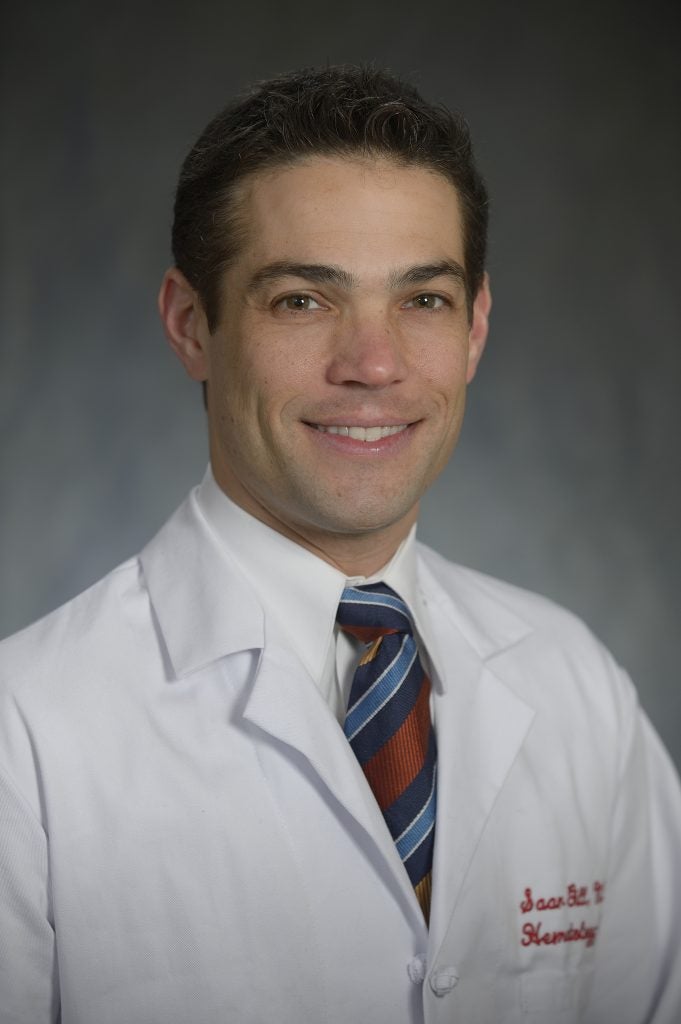This image features a professionally posed headshot of a doctor in his late 30s to early 40s, standing against a generic gray, cloudy background. The doctor is a white man with short, dark brown hair, dark brown eyebrows, and brown eyes. He is smiling directly at the camera. He is dressed in a white lab coat that is buttoned at the top, showing a white collared shirt underneath. Prominently displayed is his striped tie, featuring alternating patterns of navy blue, light blue, dark red, gold, and maroon. The lab coat has an embroidered name in red thread on the pocket, though only part of it is legible, appearing to say “San something hematology,” with a possible last name of Kennedy. This tightly cropped portrait captures him from the chest up, emphasizing his professional appearance and warm demeanor.